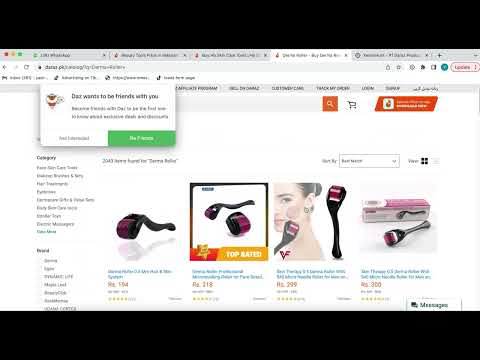The image is a screenshot of a webpage displayed in a computer browser. The browser's banner at the top is grey, indicating an active session with four open tabs lined up horizontally; the third tab from the left is currently highlighted. Below the tabs, a search bar occupies a prominent position, complete with various icons on the right-hand side. A small, white pop-up box intrudes upon the main content, featuring black text and two rectangular buttons at the bottom. The button on the left is white, while the button on the right stands out in green. The text within the pop-up is notably small.

Further down, the webpage itself presents another search bar, distinguished by an orange magnifying glass icon on the right, next to a black car icon, followed by an orange banner with white lettering. On the left side, product categories are neatly listed, while the bottom section showcases a series of products with accompanying thumbnails. Among these products, micro-needling facial rollers are distinctly visible. The screenshot is framed by black banners both at the top and bottom edges, adding contrast to the overall layout.